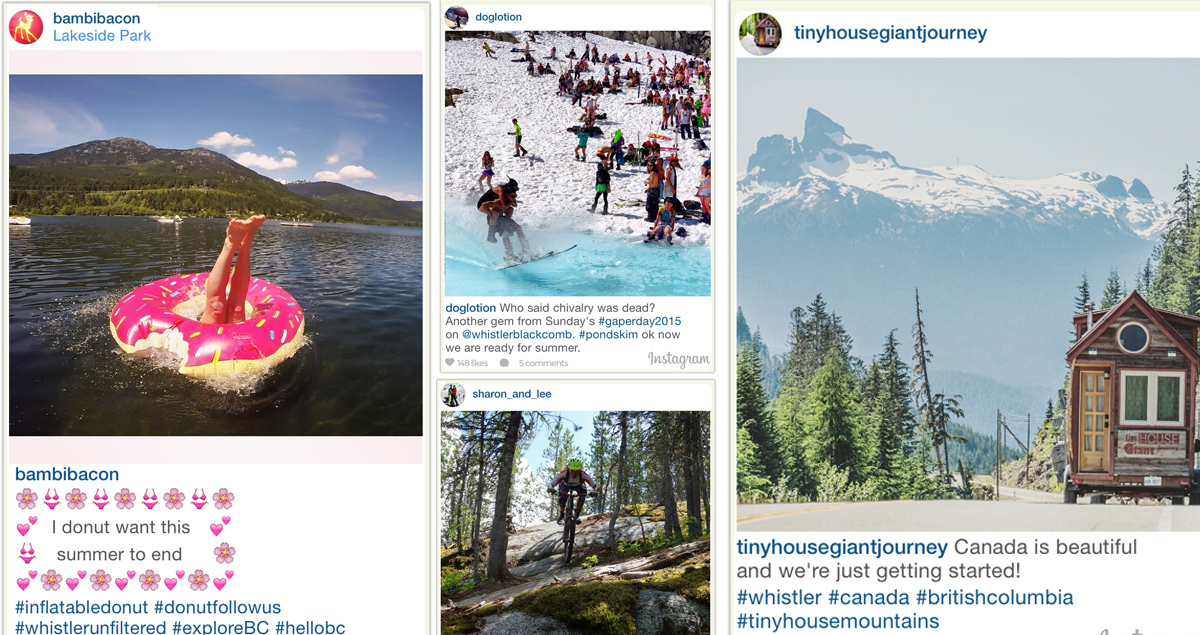This composite image resembles a collection of social media posts, each portraying vibrant scenes and adventurous moments. 

- On the far left, there's a stunning photograph of a picturesque lake with majestic mountains in the background. A vibrant pink doughnut-shaped raft with sprinkles floats on the water, from which a pair of a woman's legs protrude. The photo is attributed to a user named "Bambi Bacon" who geo-tagged their location as Lakeside Park. The whimsical caption reads, "I doughnut want this summer to end."

- In the center, two images are stacked vertically. The top image, from the user "Dog Lotion," captures the exhilaration of water skiing at a beach. Their caption playfully declares, "Who said chivalry was dead? Another gem from Sunday's Gaper Day 2015 at Whistler Blackcomb Pond Skim. Okay, now we are ready for summer." Below it, a dynamic image of mountain biking on a rugged trail is shared by "Sharon_And_Lee."

- On the far right, a serene snapshot of a tiny house nestled amidst a lush forest is seen. The user "Tiny House Giant Journey" proudly captions their photo, "Canada is beautiful, and we're just getting started."

Together, these images create a captivating mosaic of outdoor fun and scenic beauty, reflecting the diverse adventures people enjoy and share on social media.